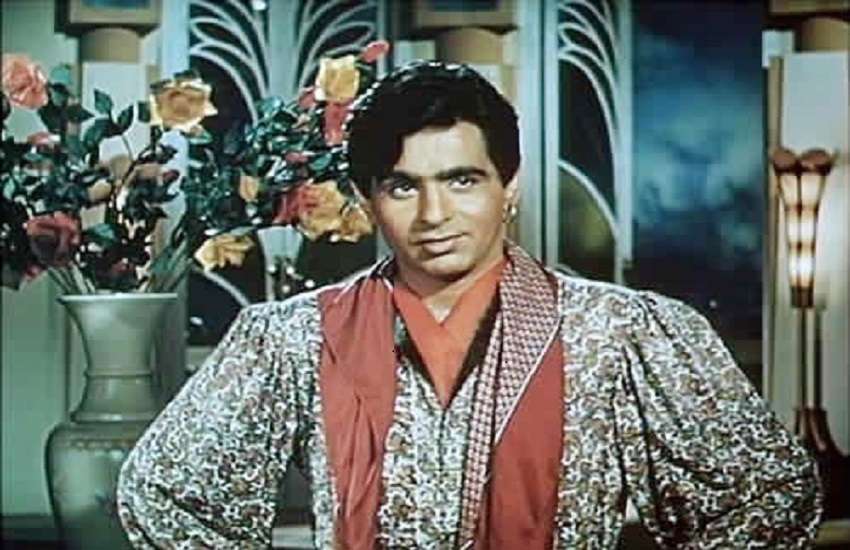This photograph features a meticulously groomed South Asian man, likely a Bollywood actor, standing in a cinematic setting. He is dressed in an ornate, exuberantly patterned shirt that is puffy at the shoulders and biceps, predominantly brown and white with intricate designs. A vivid red scarf drapes around his neck, complemented by what appears to be a secondary red fabric extending in a V-shape towards his navel. His jet-black hair is neatly styled, and he is clean-shaven, enhancing his polished appearance. He wears a gold earring in his left ear, adding a touch of flair to his look.

The background is rich with decorative elements: to his left, there are two large white containers holding a mix of artificial flowers, primarily orange, pink, and yellow roses. A bronze lantern with a vertical light and brass trim extends upwards from the floor, casting a warm glow. Behind him, various patterns adorn the wall, creating a tapestry of intricate designs. There are also hints of pillars and a doorway with colored glass panels in shades of dark and light green, adding depth and a touch of regality to the scene. The man appears posed and is looking slightly to his left, giving the impression of a staged publicity photo, possibly for a film. His entire demeanor, from the ornate costume to the elaborate set, suggests a festive, theatrical ambiance.